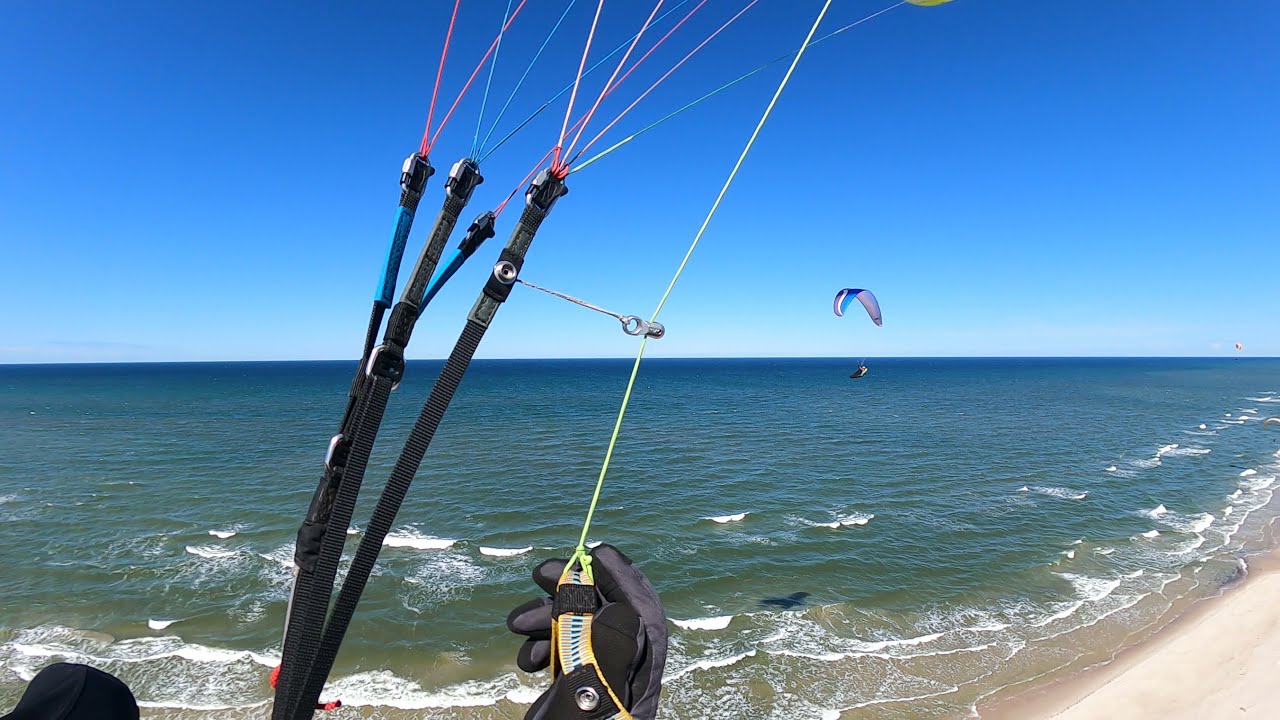The image captures a thrilling scene where the viewer's perspective is from someone who is actively parasailing over a vast expanse of water. In the foreground, the ropes and straps attached to the person's harness are clearly visible, with a gloved hand gripping one of the ropes appearing in the lower middle section of the frame. To the bottom left, a hint of a knee can be seen, further emphasizing the parasailor's presence.

The background showcases a broad, vibrant seascape. The waters are a mix of blue and green shades, with foamy white waves breaking across the scene and the blue horizon extending outward. The tranquil sky above spans a spectrum from light blue near the horizon to a deeper blue at the top, taking up about half of the image.

In the bottom right corner, there is a small section of white, sandy beach, contrasting with the surrounding water. Near the center-right area of the photo, another parasailor is visible, soaring with their parachute above the waves. The scene lacks any visible boats, suggesting that the parasailing may be occurring independent of any direct boat tow, adding to the sense of adventure and solitary excitement.